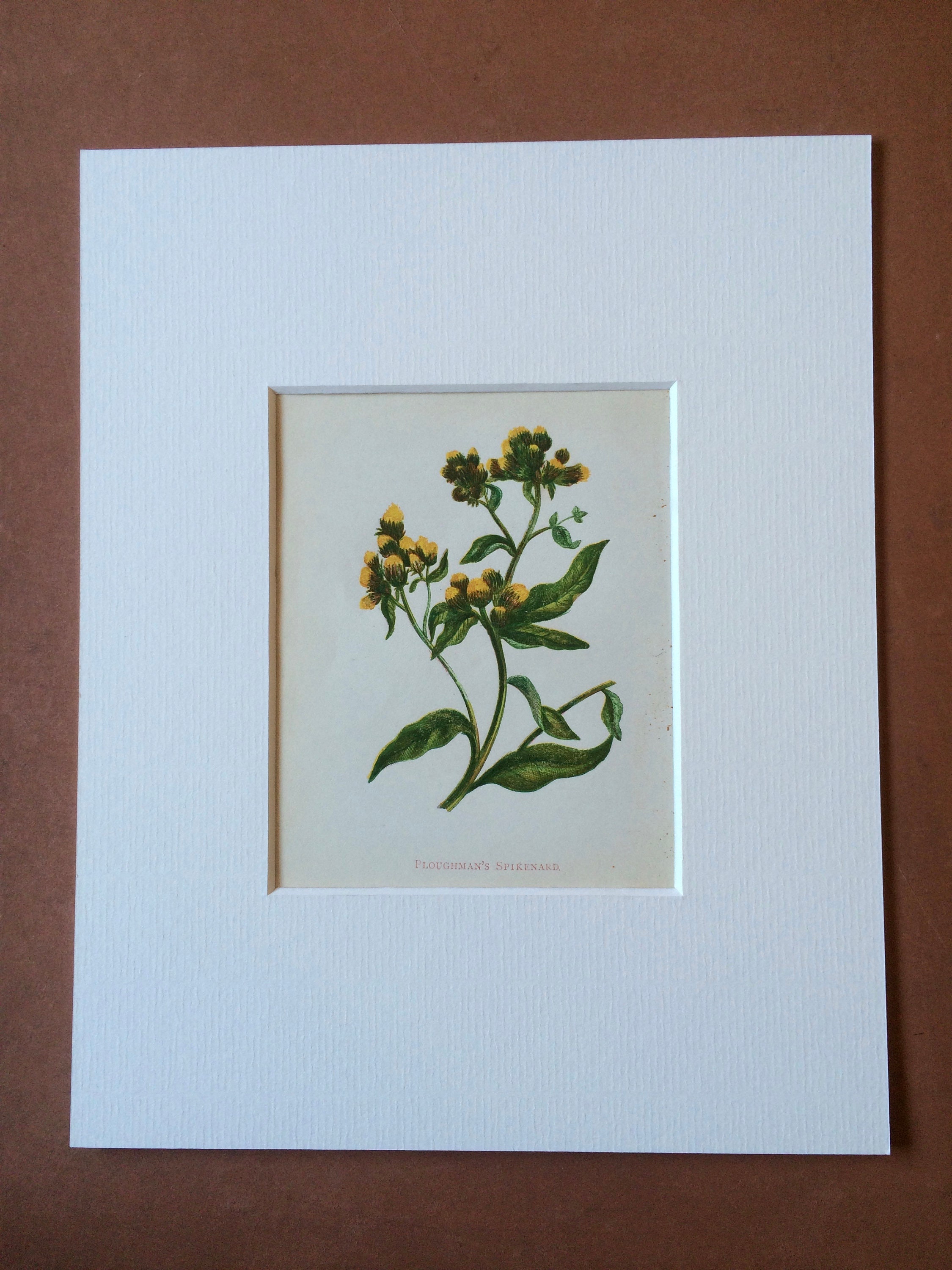This photograph, taken in portrait orientation, showcases a beautifully framed botanical painting that exudes 19th-century charm. At the center of the composition is the painting itself, displayed on a light parchment or eggshell white background. This painting illustrates a detailed plant with a gracefully curved green stem, accompanied by dark green leaves. Clusters of small, rounded yellow buds are noticeable near the center, top, and left side, suggesting the flowers have not fully bloomed.

The artwork is bordered by a wide, textured, light gray or light blue matting, which adds a subtle elegance to the presentation. Surrounding this matting is a double matting of brown textured material, providing additional depth and a rich contrast against the lighter inner layers.

The entire assembly is set against a vertically aligned brick red background, which enhances the color palette of the artwork and its frame. At the bottom of the painting, gray text is visible, likely denoting the Latin genus of the plant depicted. This image combines elements of photographic realism and representational art, capturing the timeless beauty of botanical subjects.